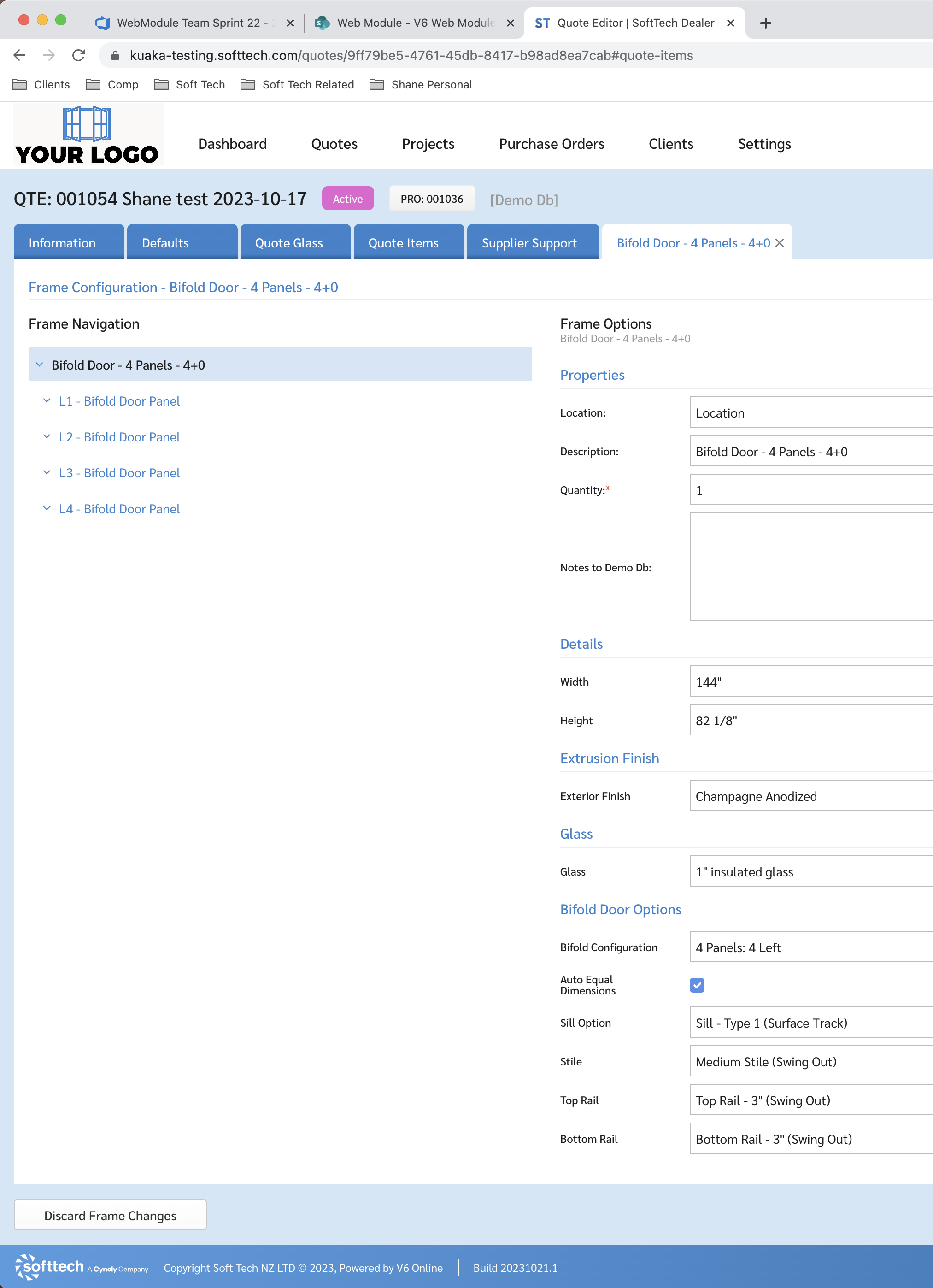This is a highly detailed caption for an image that appears to be a vertical screenshot of a desktop interface. 

---

The screenshot portrays the interface of a desktop application, structured vertically. At the top of the main page, a logo resembling either an open book or a window prominently appears, alongside navigational headers that read: Dashboard, Quotes, Projects, Purchase Orders, Clients, and Storage. Above this section lies a bookmarks toolbar, an address bar, and three tabs encased within a gray banner.

Beneath the logo, a blue banner showcases the label "QTE 001054 Shane Test 2023-10-17," accompanied by an active icon and "Pro 001036." Below this banner are five navigational tabs titled: Information, Defaults, Quote Glass, Quote Items, Supplier Support, and Bifold Door/Four Panels, with the "Bifold Door/Four Panels" tab currently selected.

To the left side of the image, there is a section devoted to Frame Configuration and Frame Navigation, featuring a dropdown menu specific to the bifold door with four panels.

The right-hand side of the screenshot displays various frame options grouped into four sections. The sections contain text boxes labeled as follows:
- **Properties**: Includes subheadings for Location, Description, Quantity, and Notes to Demo.
- **Details**: Specifies the Width and Height.
- **Extrusion Finish**: Details the Exterior Finish.
- **Glass**: Covers aspects related to glass.
- **Bifold Door Options**: Lists subcategories such as Bifold Configuration, Auto Equal Dimensions, Sill Option, STLIE, Top Rail, and Bottom Rail.

At the bottom of the interface, a dual-toned banner (light blue and medium blue) spans across the footer. The bottom-left corner features a button labeled "Discard Frame Changes." The company’s logo, labeled as "Soft Tech," is positioned on the lower left, accompanied by additional text describing company details, including the copyright information and bill number.

---

This detailed description captures the various elements and layout of the desktop application interface displayed in the screenshot.